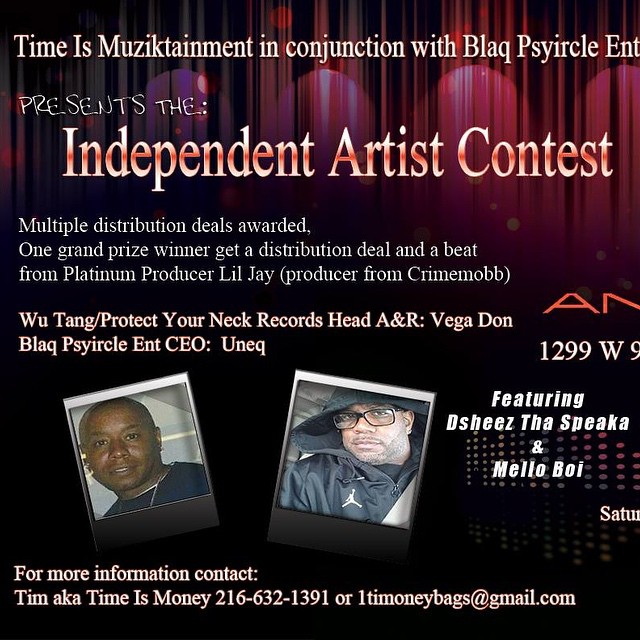The flyer advertises an upcoming Independent Artist Contest, featuring a striking visual design. The background is predominantly dark, with the bottom in black and the top adorned with a dramatic red and purple curtain lit by white spotlights. At the top, in prominent white letters, it reads: "Time is Musictainment in conjunction with Black Circle Entertainment presents the Independent Artist Contest." Below, the text elaborates: "Multiple distribution deals awarded. One grand prize winner gets a distribution deal and a beat from Platinum producer Lil Jay, from Crime Mob. Wu-Tang, Protect Your Neck Records Head A&R Vega Dawn, and Black Circle Entertainment CEO Unique."

Highlighted beneath this, there are two photographs of men involved in the event. The man on the left is a Black male, and the man on the right, also Black, wears glasses and a black windbreaker featuring a Michael Jordan logo. The lower section of the flyer mentions: "For more information, contact Tim aka Time is Money at 1tmoneybags@gmail.com" along with a phone number. The flyer also features the names "Dee Sheets the speaker" and "Mellow Boy." There's a possibility of an additional address on the right side that is partially cut off.